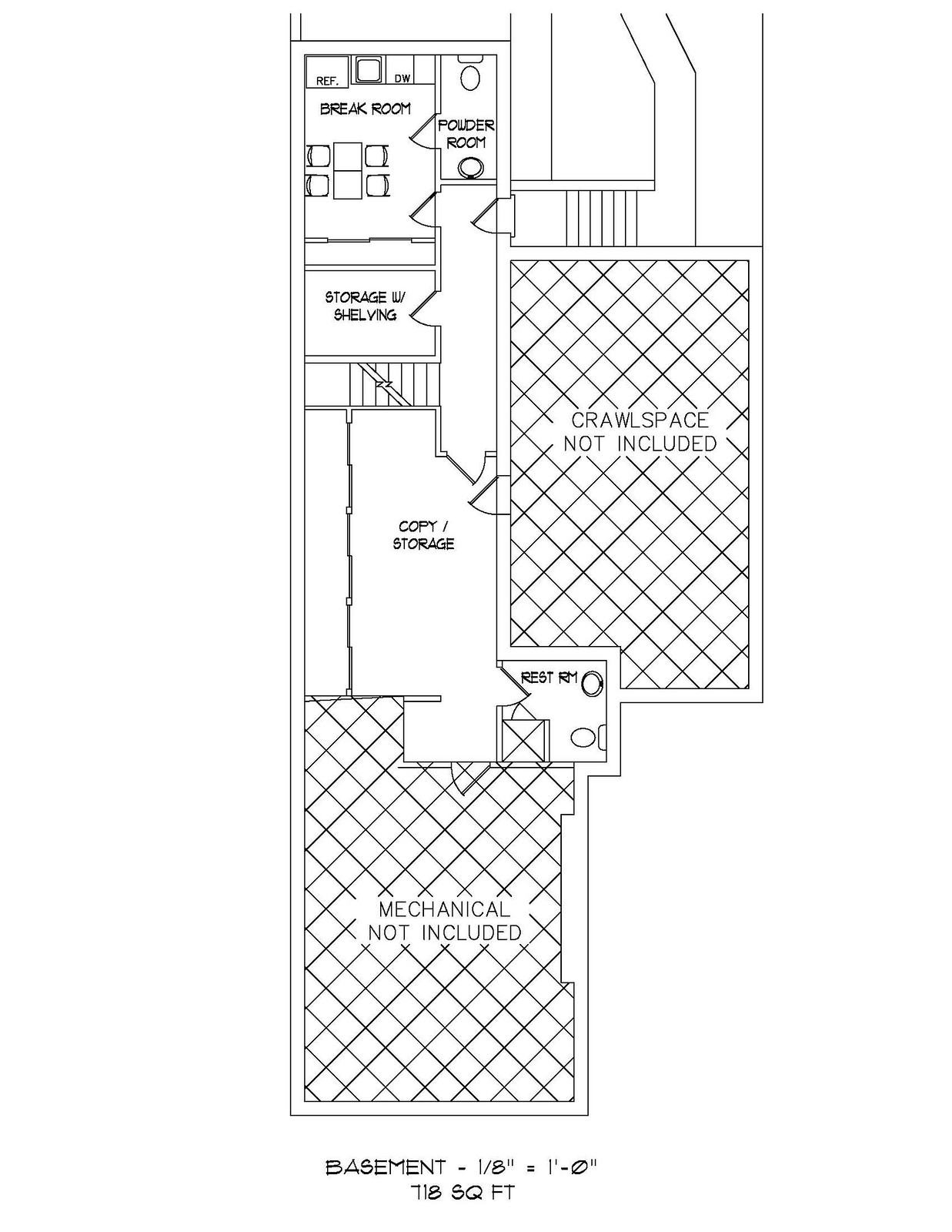This detailed caption is for an image displaying a blueprint of a work-oriented basement area:

"The blueprint illustrates a multi-functional basement layout with a total estimated area of 718 square feet, excluding the mechanical and crawl space areas. The space includes various designated rooms: at the top is the break room, centrally located is a combined coffee and storage area, and a storage and shelving room situated adjacent. There are two bathrooms—a powder room and a standard restroom. The left side features a long room extending horizontally, while to the right, there is a crawl space area. Additionally, a mechanical area is marked 'not included' in the square footage calculation. Two staircases are depicted, accessible through doorways. This blueprint appears to be designed for an office or working area within a basement space, providing essential amenities for functionality and convenience."